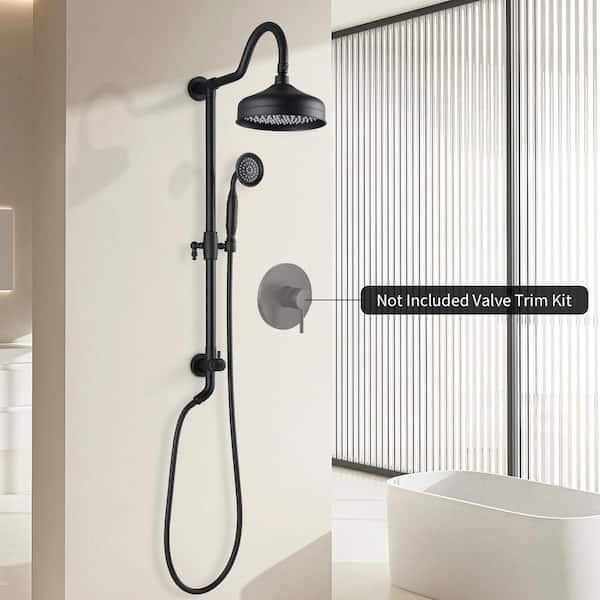The image depicts a modern bathroom centered around a black, semi-gloss rain shower head mounted to the wall, which has an ornate design. The shower head is designed to cascade water directly downward, creating a waterfall effect. There is also a detachable hand-held shower head with a hose that attaches to an adjustable clamp on a wall-mounted pole, offering flexibility and control. Below the shower assembly is a gray disc acting as the control panel for adjusting water temperature and flow. A note indicates that the valve trim kit for this control panel is not included. The bathroom features a sleek, white standalone bathtub on a white floor. The walls are also white, with a 30-degree angled wall to the left and privacy glass sliding doors in the background. There is a window behind the bathtub, covered by blinds. The décor is minimal, focusing solely on the essential fixtures.